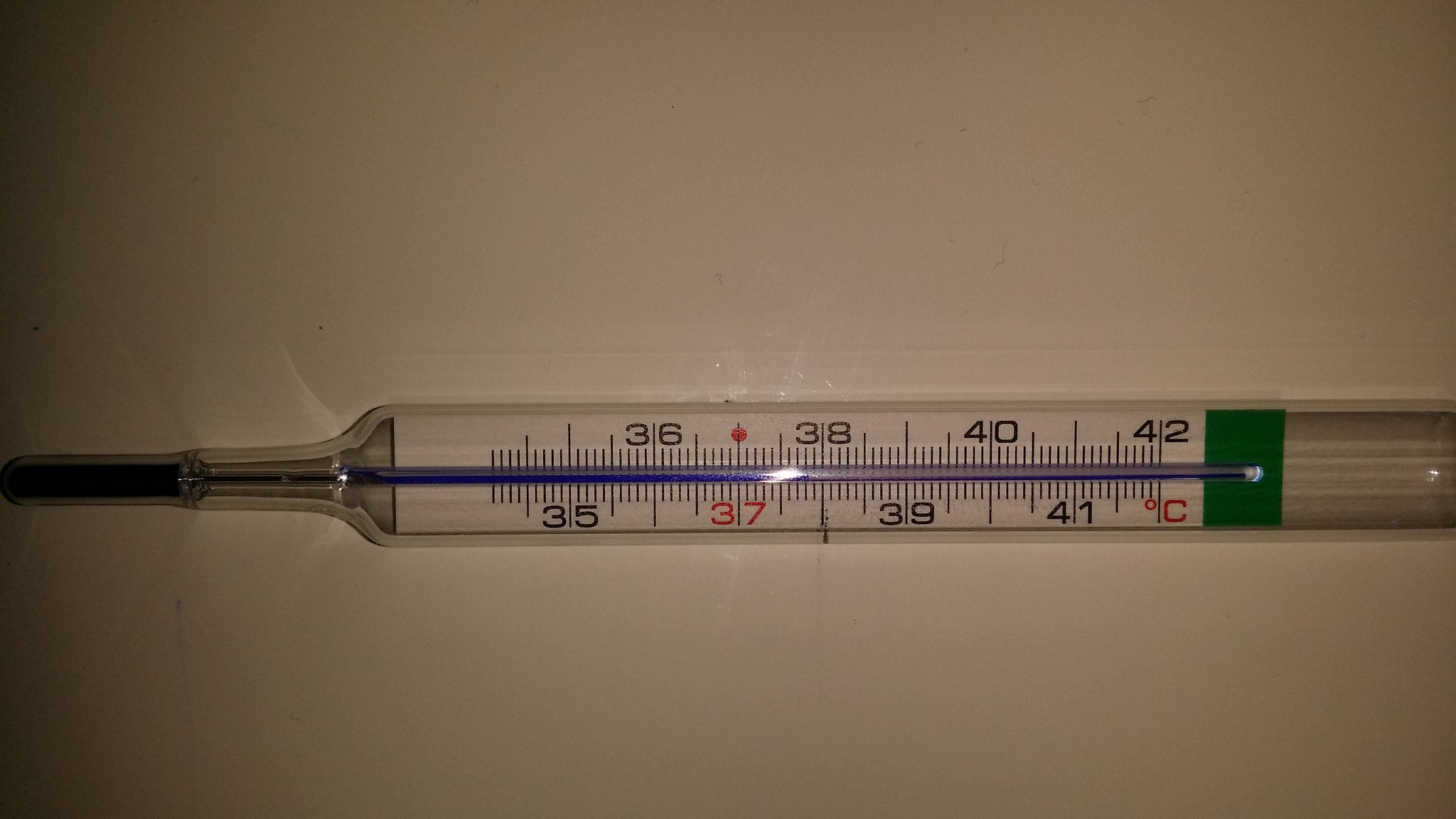This horizontal color photograph features a detailed view of a temperature gauge or thermometer, calibrated in Celsius. The gauge is positioned horizontally, revealing two sets of numbers: the top sequence displays 36, 38, 40, and 42, while the bottom sequence shows 35, 37, 39, and 41. The temperature range on the scale extends from 35°C to 42°C, though the device could potentially register temperatures slightly lower, possibly down to 34°C, despite the absence of this number on the gauge. A notable red dot marks the 37°C indicator. The thermometer appears encased in either plastic or glass, with one end tapered and somewhat sharp, suitable for insertion into a mouth, soil, or another medium, and a flattened opposite end designed for easy handling or hanging. The partial view of the image leaves the specific application of the thermometer—whether for human use or environmental measurement—ambiguous.